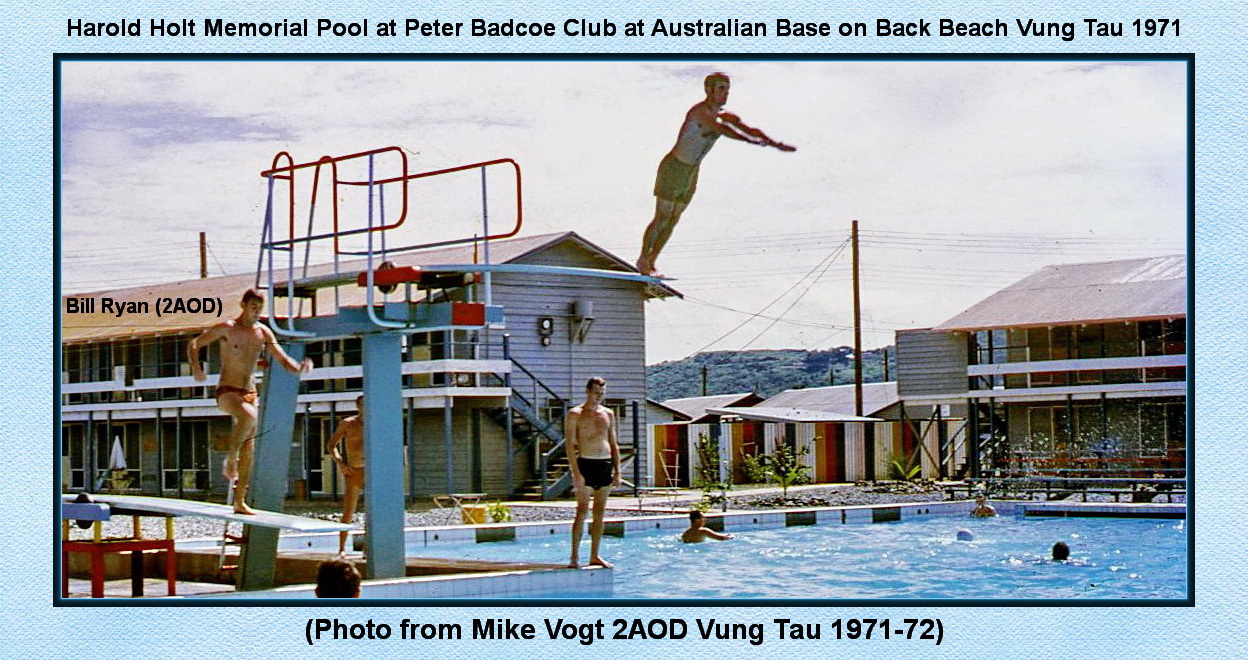In this vivid full-color photograph, we see a lively pool scene under the bright daylight at the Harold Holt Memorial Pool, located at the Peter Badko Club within the Australian Base on Back Beach, Vung Tau, Vietnam, circa 1971. The image captures a dynamic moment: a man in red or reddish-brown bathing trunks is mid-air, diving off a high board, while another is in motion, running down a lower diving board, preparing to leap. Several men are swimming in the pool, while a few others stand by the poolside. A beach volleyball or water polo ball floats on the water’s surface. In the background, the two-story dormitories hint at the militaristic setting, likely housing troops during the Vietnam War. The scenic backdrop of low hills covered with scrub bushes adds a picturesque touch reminiscent of landscapes from the TV show MASH. The photograph, enclosed in a light blue bordered box, is credited to Mike Vogt of 2AOD, and also mentions Bill Ryan, suggesting he might be the person diving off the low board. This historical snapshot provides a glimpse into the leisure moments of soldiers amidst the backdrop of the Vietnam War.